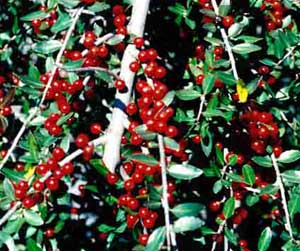This square-shaped, vintage color photograph, likely taken on a film camera from the 1980s, features a close-up of an array of vibrant red berries clustered along slender white branches of a bush or small tree. Extending from a central thin branch, multiple smaller branches are adorned with oval-shaped, green leaves streaked with a thin green line, as well as some yellow leaves. The berries, possibly of a holly plant, stand out brightly against a backdrop of green, though the overall image's color saturation appears slightly washed out due to the bright sunlight under which it was taken. Despite the image’s age and lower quality, the contrasting colors of the red berries and green foliage remain striking. The photograph is small and lacks any text, focusing solely on the dense, downward-growing branches, through which no background is visible. The vibrant red berries, reminiscent of holly, provide eye-catching details that suggest both the beauty and possibly the danger of the small, round fruits. One leaf among this carefully arranged foliage stands out with a distinct lime-green hue, adding an intriguing touch to the otherwise harmonious color palette.